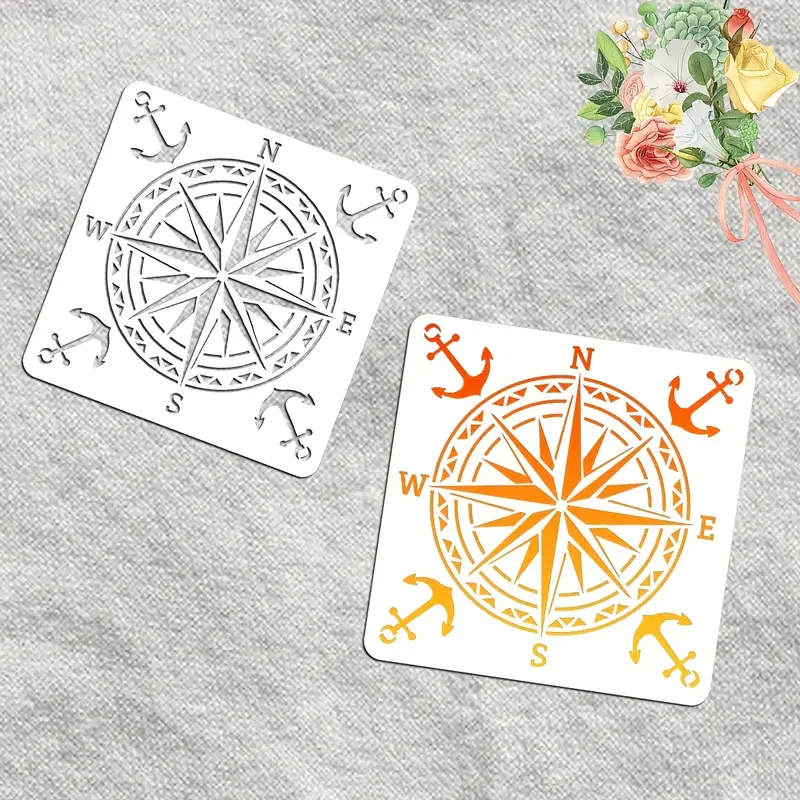This image features a white tablecloth background with an array of colorful flowers tied with a pink ribbon in the upper right-hand corner, including a yellow rose, a pink rose, leafy greens, and two white petunias—one open and one closed. Centered in the composition are two compass stencils, each prominently featuring the cardinal directions North, South, East, and West, along with anchors on each corner and a compass star in the middle. The stencil on the left is a solid black and white design, while the stencil on the right displays a gradient transitioning from bright yellow to vibrant orange. Both stencils are enhanced with intricate details, such as a surrounding circle with trapezoidal shapes, creating a balanced and symmetrical visual appeal. The background of the entire scene is framed in a subtle gray.